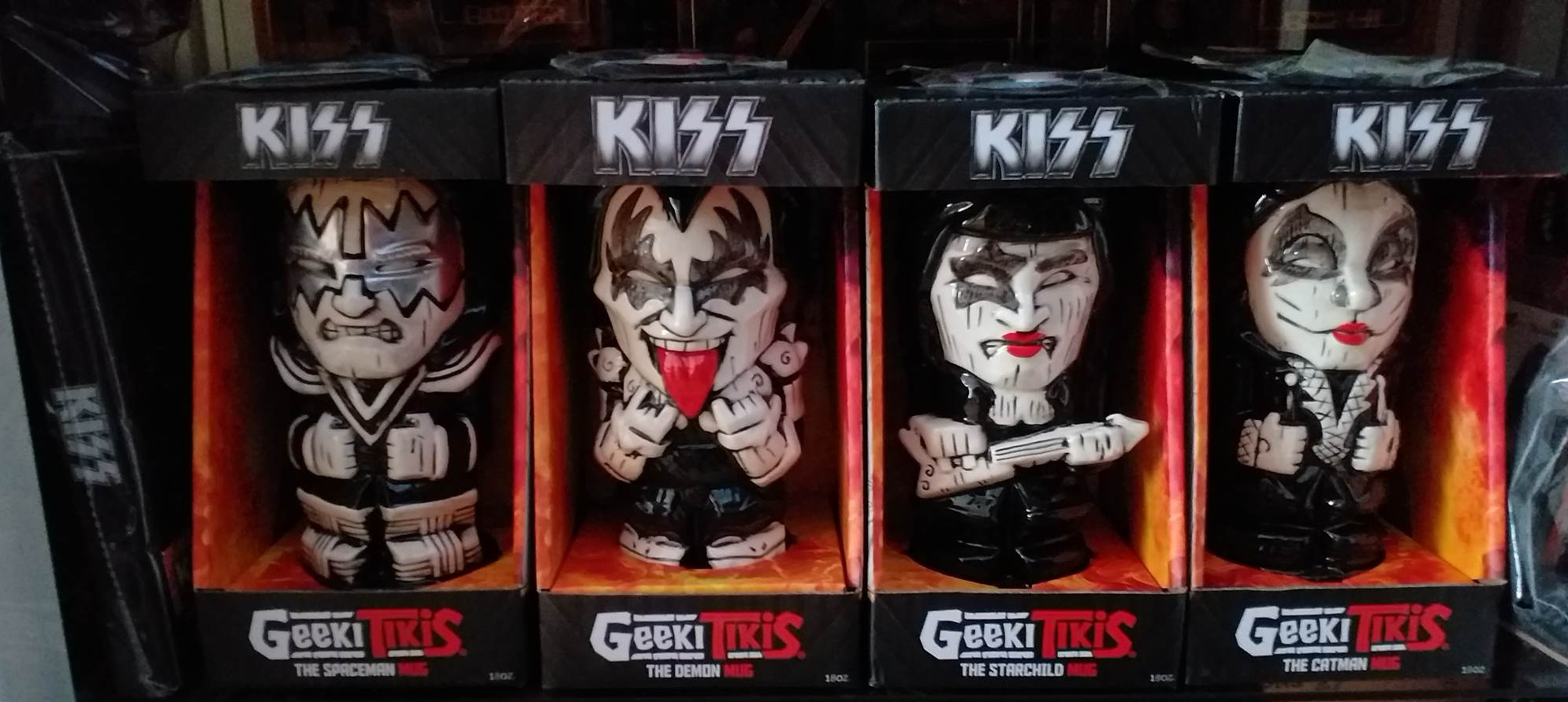This image showcases a display of four collectible KISS-themed Geeky Tikis mugs. Each mug, designed to resemble a member of the iconic rock band KISS, is encased in its own black box. The band’s name, "KISS," is prominently displayed in white text at the top of each box, while "Geeky Tikis" is written below, with "Geeky" in white and "Tikis" in red. The interior of each box features a background with red and orange flame-like designs, adding to the dramatic presentation.

The mugs portray the band members with distinctive details:
1. **The Spaceman (Ace Frehley)**: Recognizable by his silver star design around the eyes.
2. **The Demon (Gene Simmons)**: Noted for his black eye markings and a prominently stuck-out red tongue.
3. **The Starchild (Paul Stanley)**: Features a single silver star around his left eye and red lipstick.
4. **The Catman (Peter Criss)**: Has cat-like makeup with whisker details and red lipstick, bearing a feline resemblance.

Each character dons traditional KISS attire in black, white, and gray, with some variations in shoe and glove colors. The boxes are aligned neatly on what appears to be a store shelf, with hints of additional KISS merchandise visible in the corners of the image. The collective display captures the bold and theatrical essence of the band, making it a standout piece for KISS memorabilia collectors.